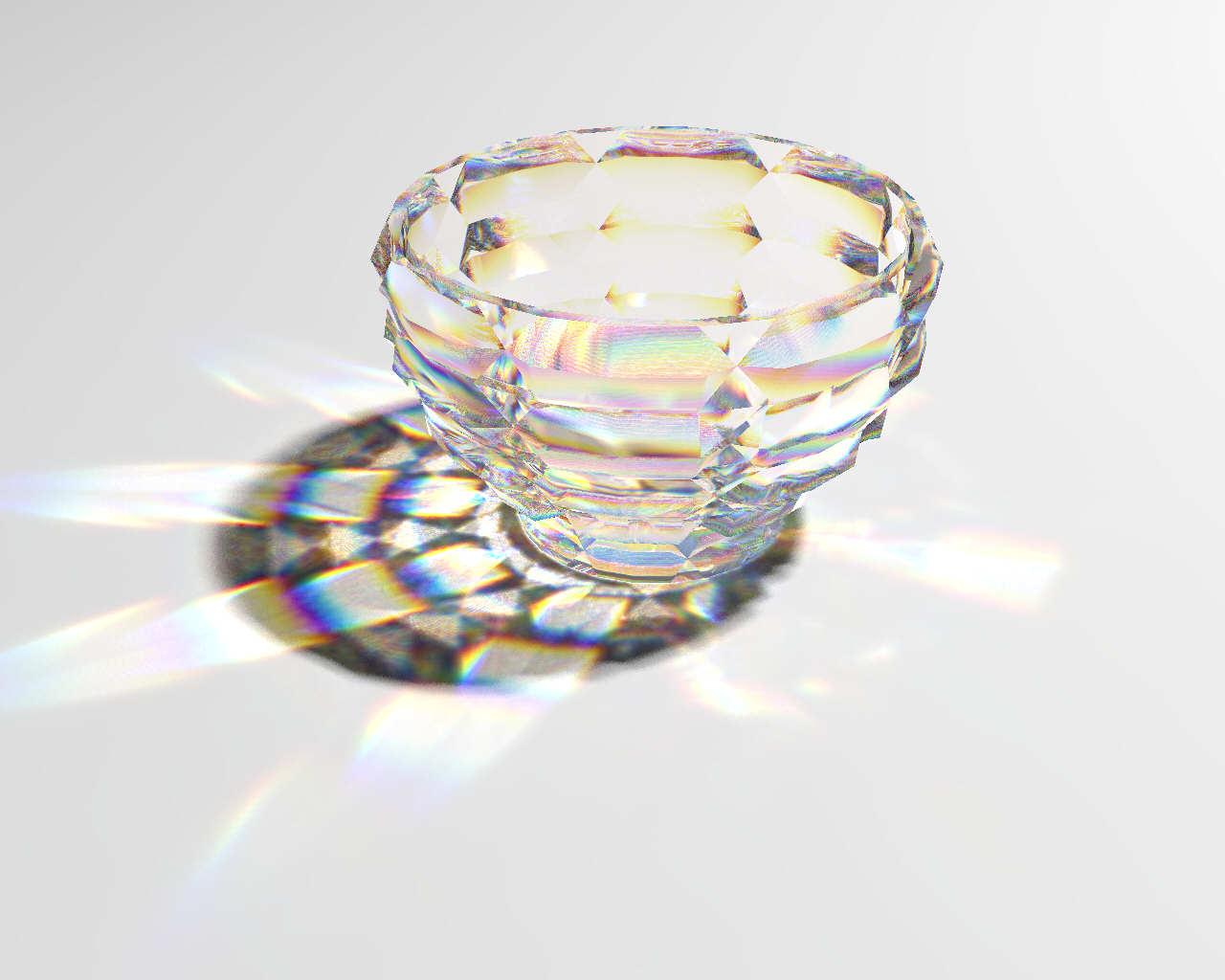This is a photograph of a small, intricate crystal bowl positioned on a light gray background. The bowl, narrow at the bottom and widening towards the top, features many facets and sections that create a prismatic effect when hit by sunlight. Rays of rainbow hues—yellow, green, and more—emanate from the bowl, casting a colorful, diffuse light onto the backdrop. The crystal bowl itself casts a gray circular shadow overlayed with lighter, colorful bands with smoothly transitioning edges. White highlights surround the bowl, emphasizing its sculpted sections and the mesmerizing play of light. The image beautifully showcases how the bowl reacts to light, displaying an array of prismatic colors and soft-edged bands that transition seamlessly, creating a stunning visual display.